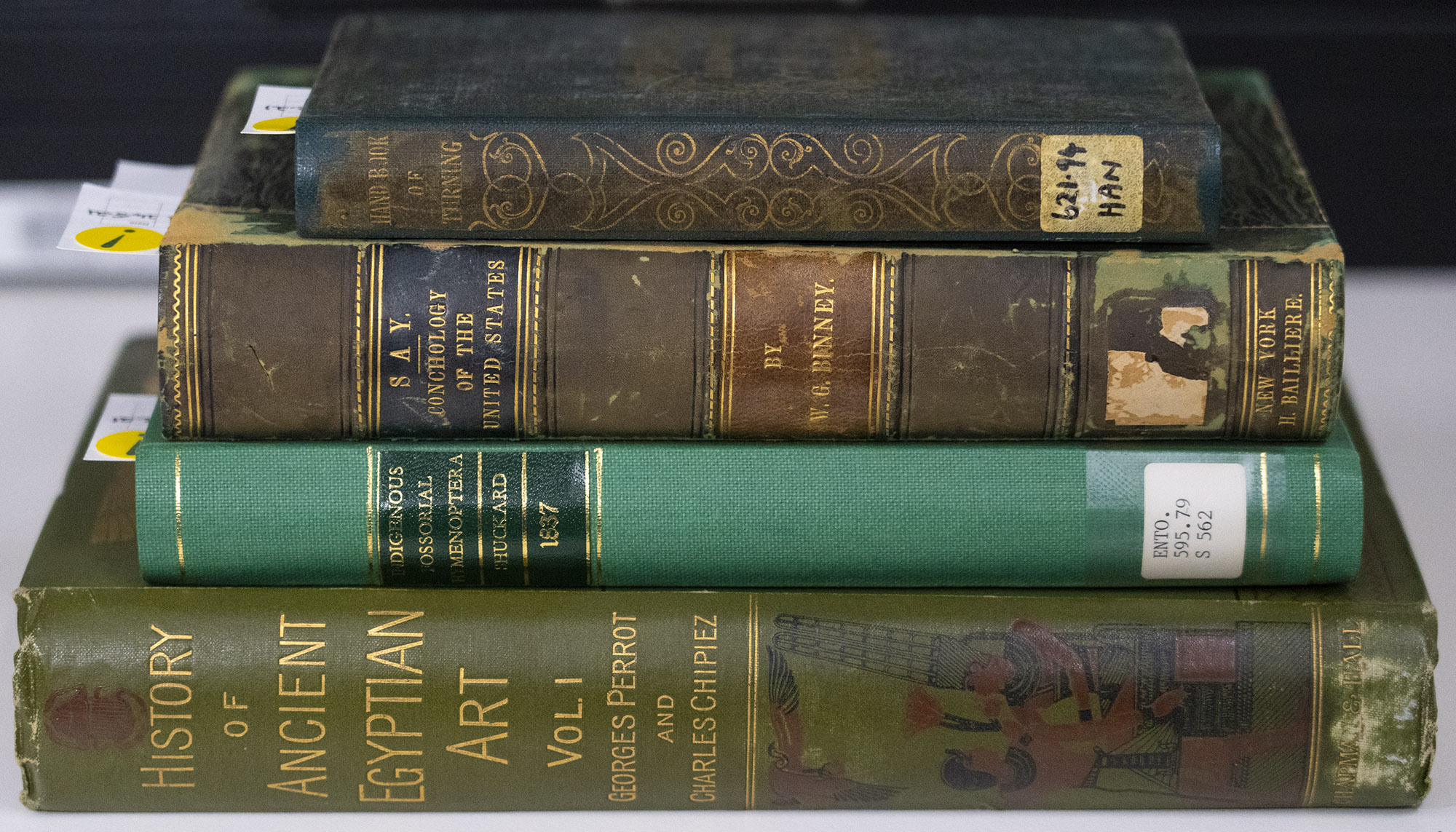This is a color photograph of a stack of four old and worn library books, arranged from largest at the bottom to smallest at the top. The bottom book, with an olive green cover, is titled "The History of Ancient Egyptian Art, Volume 1" by Georges Perrot and Charles Chipiez. Its spine features an illustration of two Egyptian figures, one with a tall hat and a servant holding a bird, and is adorned with gold type. The book shows significant wear on its edges. The second book from the bottom is bright Kelly green with gold type and bands, featuring a complex design with a black box and the year 1837. A library sticker reading 595.79S562 is located at the bottom of the spine. The third book is vintage and quite worn, with its title difficult to decipher. The smallest book at the top has a hazy title and features a beautiful gold inlay design on its spine. All but the bottom book have library cards sticking out, with visible exclamation points, suggesting they are on hold at a library.